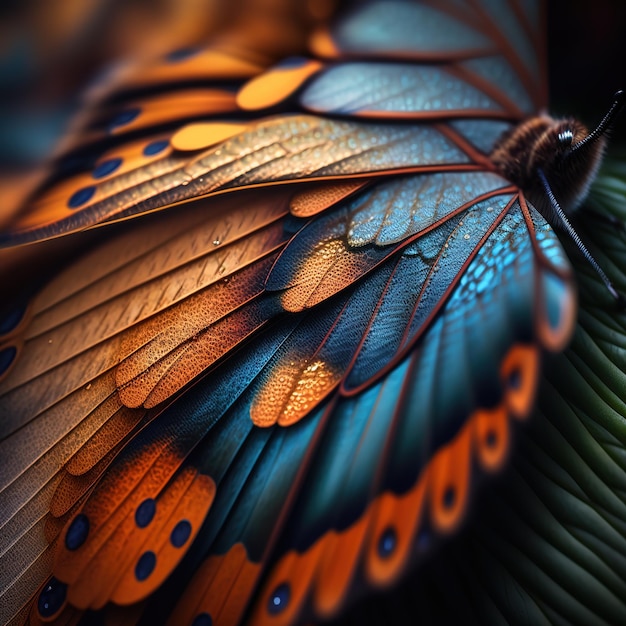This image is a detailed close-up, likely an extreme macro photograph or an AI-generated art piece, depicting a moth or butterfly. The focal subject reveals an intricate and vibrant blend of colors on its wings, primarily blue near the body, transitioning to a striking orange as they extend outwards. The wing edges are adorned with blue spots, some containing smaller white dots. The texture of the wings is delicate and slightly iridescent, showcasing individual scales. On the right, a portion of the moth's or butterfly's fuzzy head, two textured antennas, and one visible eye are discernible. Background elements include blurred green vines or leaves on the right side, contributing to a green-striped appearance. The overall image features areas of intentional blurriness, particularly towards the top left and lower right, emphasizing the main subject's beauty and texture.